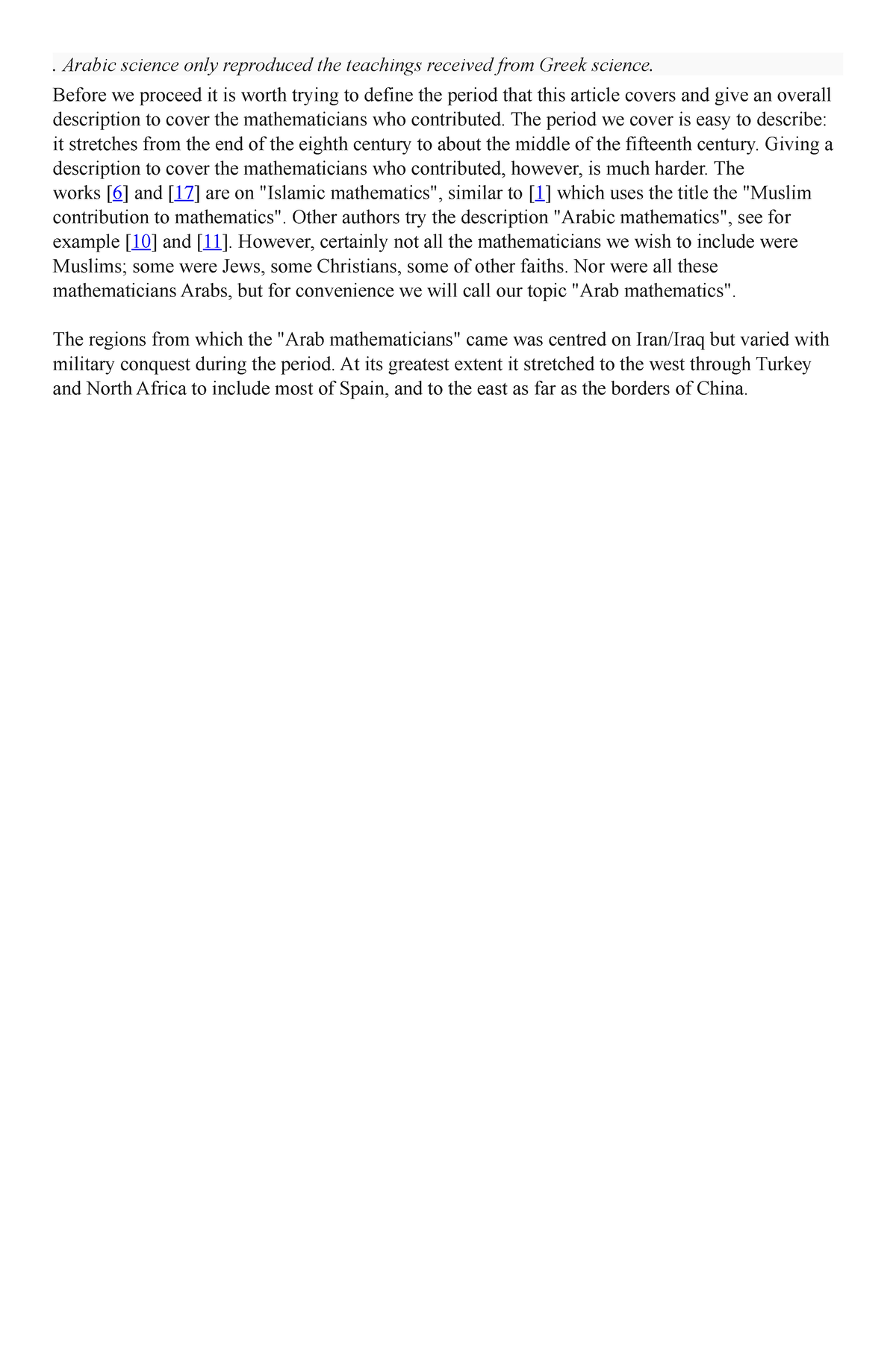This image features text discussing the scope and influence of Arabic science, particularly highlighting its role in preserving and enhancing Greek scientific teachings. The period under consideration spans from the end of the 8th century to the mid-15th century, illustrating a significant era of mathematical development. The narrative delves into the complexities of identifying and describing the contributions of mathematicians from this era. While some scholars refer to this body of work as Islamic mathematics, others prefer the term Arabic mathematics, as the contributors included not only Muslims but also Jews, Christians, and individuals of various faiths. Notable references to the topic are cited, such as those found in sources labeled 10 and 11.